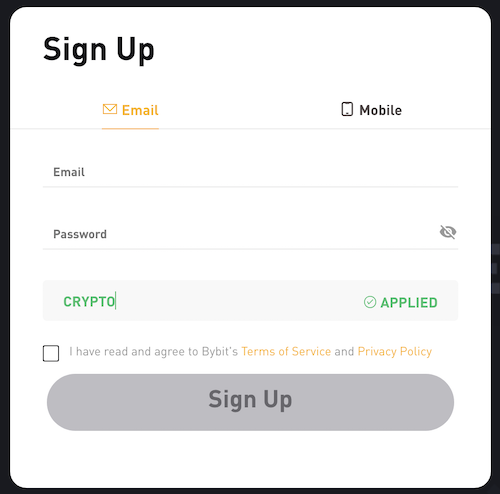The image depicts the sign-up section of a mobile phone application. At the top, there are two tabs for selecting between email and mobile number registration, with the email option highlighted in yellow, indicating it is currently chosen. Below, there are input fields for the user's email, password, and a code, which appears to be related to cryptocurrency, as the term "crypto" is mentioned. 

Next to the password field, there is an eye icon with a slash through it, signifying that the password entered will not be revealed. The section includes a checkbox with the text, "I have read and agreed to the Terms of Service and Privacy Policy," where "Terms of Service" and "Privacy Policy" are highlighted in yellow, indicating clickable hyperlinks.

The "Sign Up" button at the bottom is grayed out, suggesting that the form is incomplete or conditions have not been met for submission. This entire sign-up section is enclosed within a distinct black box for clarity and emphasis.